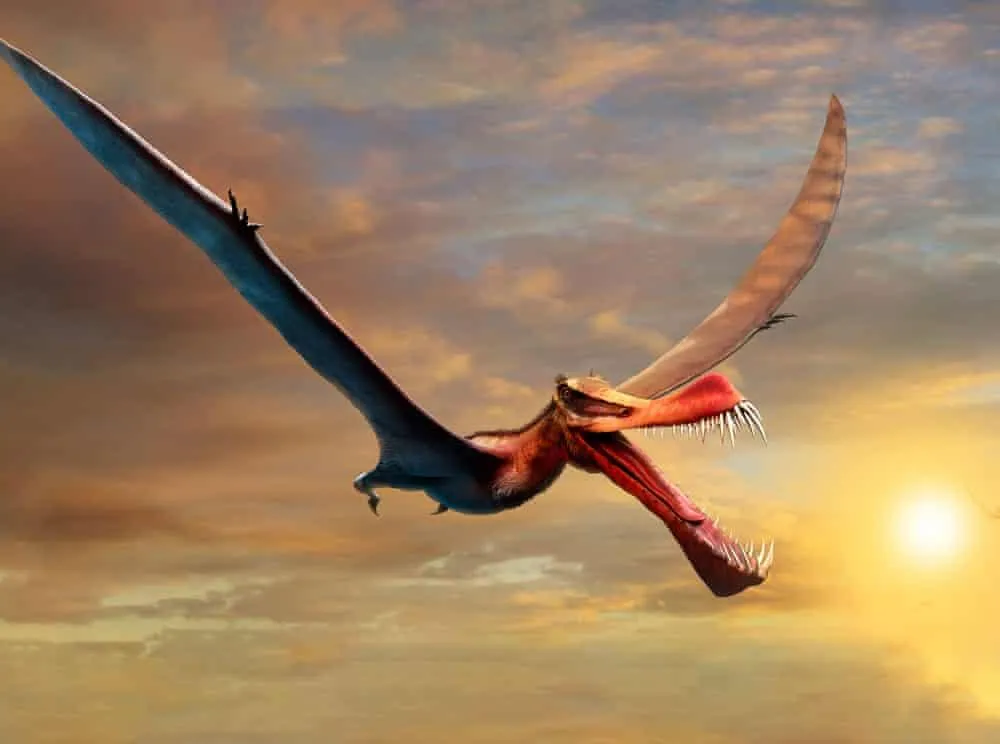The image showcases a stylized, ultimately monstrous depiction of a prehistoric bird, likely a computer-generated pterodactyl. The creature, soaring through a cloud-filled sky that transitions from shades of gray to hints of blue and white, commands attention with its immense wingspan. One of its wings displays a darker gray hue on the underside due to the sunlight's angle, while the other is slightly blue and flesh-colored with a mottled light gray on top. The menacing bird has an extraordinarily large, open mouth lined with razor-sharp teeth, which are especially prominent at the front and taper slightly towards the back. Its face and jaw are vividly red, adding to its terrifying appearance. Positioned near the middle-right of the image, the pterodactyl seems poised to consume the partially obscured sun behind it, enhancing the dramatic and eerie atmosphere of the scene. Its dangling legs and feet are clearly visible, completing this awe-inspiring and fearsome portrayal of prehistoric might.